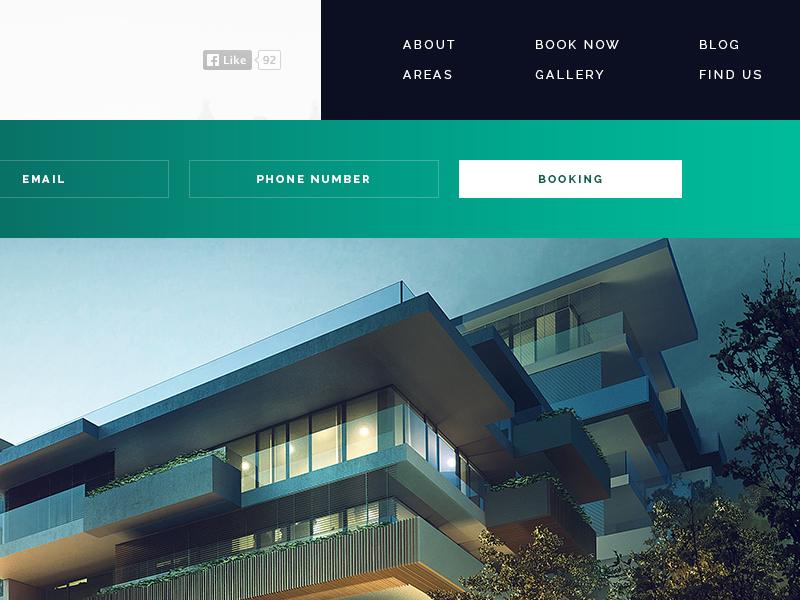The image appears to be a zoomed-in screenshot of the upper right corner of a website's navigation panel. The visible section tabs are organized horizontally from left to right. The first tab is labeled "About," followed by "Book Now," and "Blog." Below these, there are three more tabs labeled "Areas," "Gallery," and "Find Us." 

In addition to the section tabs, the left side of the image shows contact information tabs for "Email" and "Phone Number," whereas the right side features a highlighted "Booking" button. Notably, the "Booking" button is highlighted in white, contrasting with the green background of the other tabs, which seamlessly blend into the overarching banner design.

At the bottom of the image, there is a small picture depicting a house, adding a visual element to the corner of the website. The overall color theme integrates green and white, providing a cohesive look to the navigation panel.